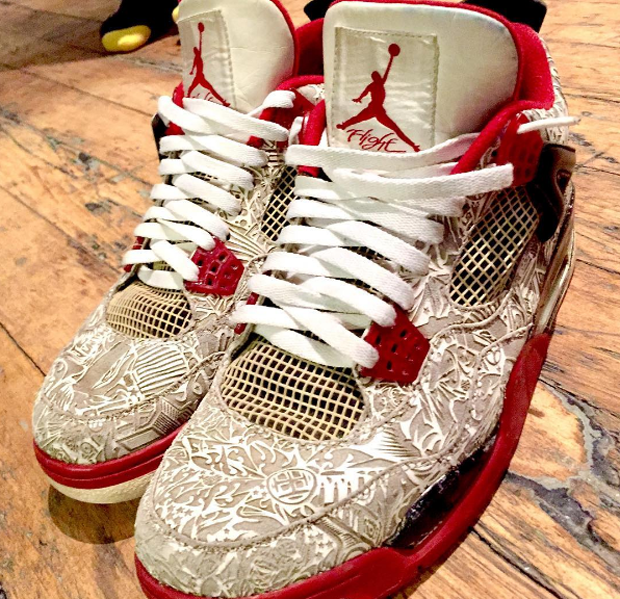In this detailed color photograph, presented in a square format, the subject is a close-up of a pair of Air Jordan 4 Retro Laser 2005 sneakers, depicted in a realistic, representational style common to product photography. These unique sports shoes, predominantly white and red, are positioned side by side on a pine hardwood floor, with the toes oriented towards the bottom left corner and the heels towards the top right. The sneakers feature a distinctive white and cream-colored brocade or tan paisley embroidery around the toe area and the sides, creating an intricate, eye-catching design.

The shoes are primarily red at the upper body, fading to the embroidered pattern near the first eyelet. The mesh inserts are visible below the lace-up area and the side panels, adding an unusual design element with netting above the toes and along the ankle area. The red soles contrast sharply with the white undersides, while the white shoelaces, only partially laced, emphasize the shoes' sporty aesthetic. The red interior lining, complete with trim around the ankle, and the white pad inside the shoe prominently display the iconic red silhouette of Michael Jordan dunking a basketball, with the word "FLIGHT" inscribed underneath.

Additionally, there's a subtle detail of a person's foot in a black-and-yellow sock visible in the upper left corner, slightly blurred, ensuring the sneakers remain the focal point of the image. This human element adds a touch of context to the composition, indicating the sneakers are new yet positioned in a real-life setting, enhancing the overall realism of the photograph.